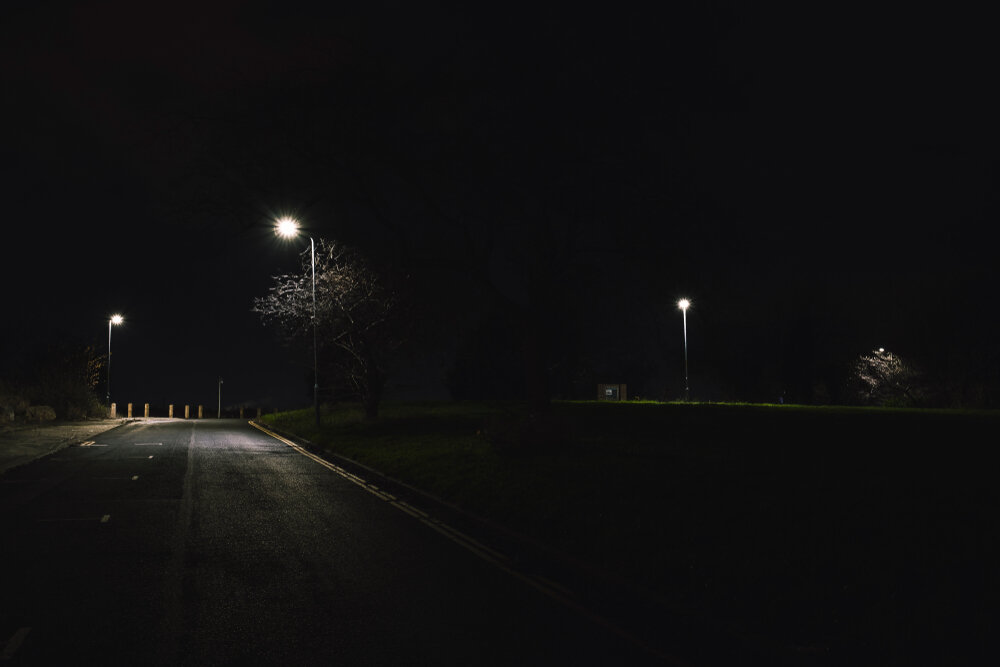The image depicts a very dark street scene shrouded in night, where intermittent street lamps cast faint pools of light amidst pervasive darkness. The barely illuminating streetlights reveal a road with dashed lines and a mix of black and gray pavement. In the distance, yellow barriers hint at a boundary or transition area.

On the right side, a small brick structure or sign is dimly visible due to a nearby street lamp, along with a bush that's similarly illuminated. The left side of the image features another street lamp at the far end, barely highlighting the street as it begins to curve.

In the forefront, a tree stands next to a street lamp, with another bush positioned on the left side, all sitting among patches of grass. Additionally, unlit lamps add to the shadows, deepening the overall sense of obscurity.

The scene's minimal lighting creates a stark contrast, revealing just enough to suggest a grassy area, potentially a park, on the right side, while the street appears more prominent on the left. The sky looms completely black overhead, intensifying the image's enveloping darkness.